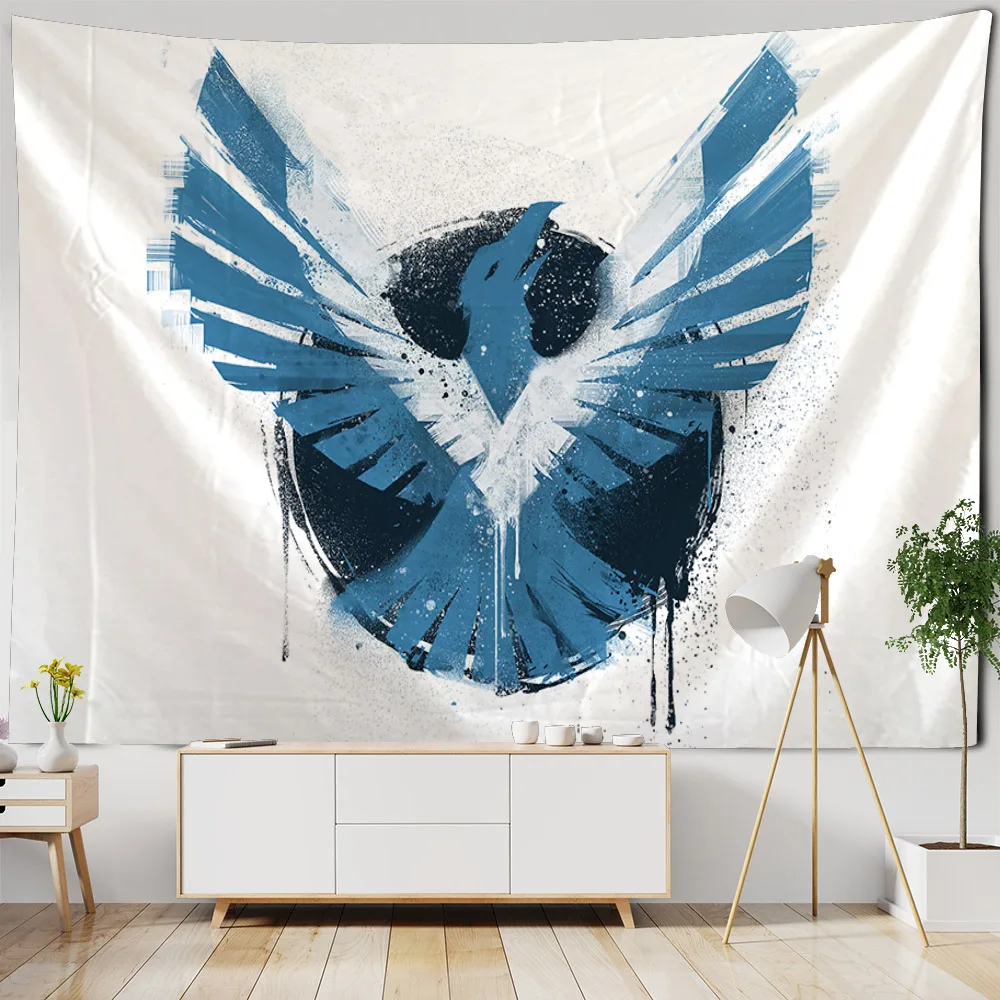The image showcases a meticulously arranged indoor room dominated by a large wall hanging. This hanging is a smooth white canvas featuring an impressive depiction of a blue bird, reminiscent of a phoenix. The bird has its wings spread high and its head held aloft. Its deep blue plumage contrasts sharply with a white V-shaped marking around its neck and additional white tinges at the wing tips. Behind the bird is a dark navy blue circle, emphasizing its form. The canvas is slightly curved at the top corners, giving it a natural drape effect.

The room's design is equally detailed. The floor is covered with light beige wooden panels that add warmth to the space. Centered against the wall is a long, rectangular white cabinet with two drawers. Atop the cabinet, there's a variety of objects: cups on the right side, a book on the top left, and other miscellaneous items. To the left of this cabinet stands a small table or nightstand holding a white square pot with a small green plant, featuring yellow petals.

To the right of the cabinet, a tall tripod stand supports a white light. Adjacent to this stand is another plant in a similarly white square pot, matching the height of the light. The gray wall behind these furnishings contrasts harmoniously with the wooden flooring, bringing cohesiveness to the entire setup.